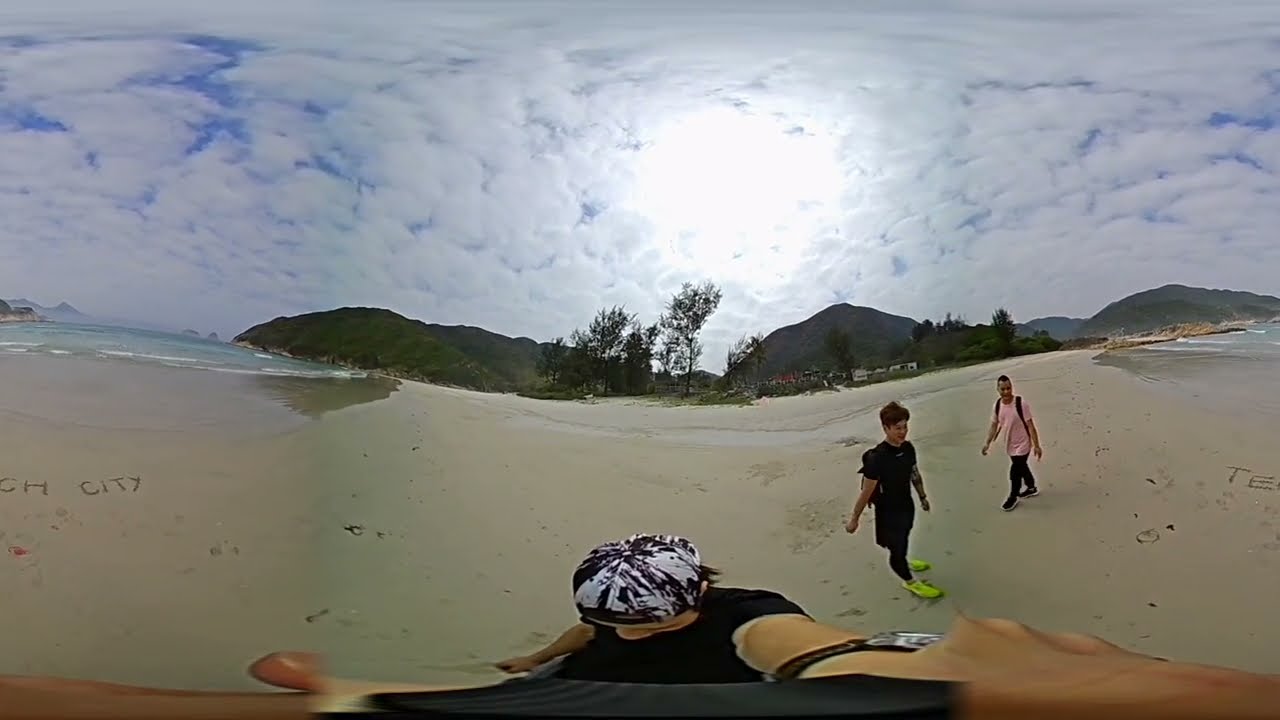The distorted fisheye lens image portrays a scenic beach with a muddy, light gray expanse stretching across the center and water approaching from both sides. Central to the image is a Caucasian man, wearing a black shirt and a white and gold cap backwards. He sports a wristwatch on his right wrist and appears to be holding the camera. 

To his right, two young men walk along the beach. The first man, in a black short-sleeved shirt and black pants, has light green shoes and a backpack. He has black hair and walks beside another man in a pink shirt and dark pants, also carrying a backpack. This second man faces rightwards. 

The backdrop features a row of rolling, shadowed hills beneath a mostly cloudy sky, with pockets of blue and an intense, bright light like the sun trying to break through in the center. Lush, large trees with green leaves dot the hilly landscape. Faint etchings in the sand spell out "Tech City," and houses are visible between the trees and the hills.